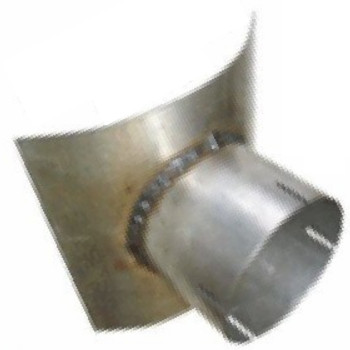The photograph shows a blurry, heavily pixelated image of a metal component, suggesting it has either been heavily edited or saved repeatedly, resulting in diminished quality. The item appears to float in a white void due to the stark white background. The main object is a curved piece of metal, with the curve oriented toward the top left of the image. Attached to this curved metal piece is a small, wide cylinder featuring four slits or notches near its edge. This cylinder is welded onto the curved section, with the weld appearing very dark or blackened, indicating burning. The metal around the weld also shows various brown spots, suggesting weathering or rust. The curved metal piece itself is a darker, weathered silver, contrasting with the blackened welding marks, adding to its rugged, industrial appearance.